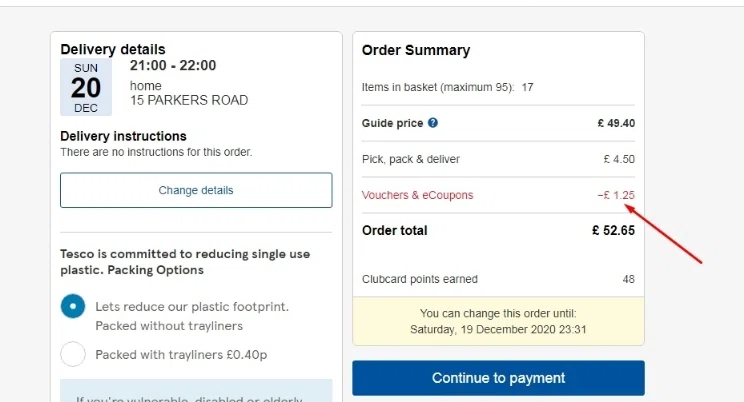This image displays two screenshots of an order confirmation and details, positioned side by side within a grayish box. The screenshots provide comprehensive information about the delivery and order summary.

On the left side, the first screenshot contains the delivery details and additional information as follows:
- **Delivery Details:** Scheduled for Sunday, 20th of December, between 21:00 and 22:00, to the address 15 Parkers Road.
- **Delivery Instructions:** None specified for this order.
- There is a blue button labeled "Change Details."
- **Environmental Message:** Tesco is committed to reducing single-use plastics. Options are:
  - **Packed Without Tray Liners:** Indicated by a blue bullet point.
  - **Packed With Tray Liners:** An additional cost of £0.40, indicated by an open bullet point.
- Below this section, there is a partially visible blue box with text that is cut off, making the content unreadable.

On the right side, the second screenshot provides an order summary:
- **Order Summary:**
  - **Items in Basket:** Maximum allowed is 95, with the current count at 17.
  - **Guide Price:** Listed as £49.40, denoted with a question mark in a blue circle.
  - **Pick, Pack, and Deliver Fee:** £4.50.
  - **Vouchers and E-Coupons:** Applied discount of -£1.25.
  - **Order Total:** £52.65.
- **Club Card Points Earned:** 48 points.
- **Order Modification Notice:** The order can be changed until Saturday, 19th December 2020, at 23:31.
- Below this notice, there is a yellow box with the aforementioned modification details, and a blue button that says "Continue to Payment."